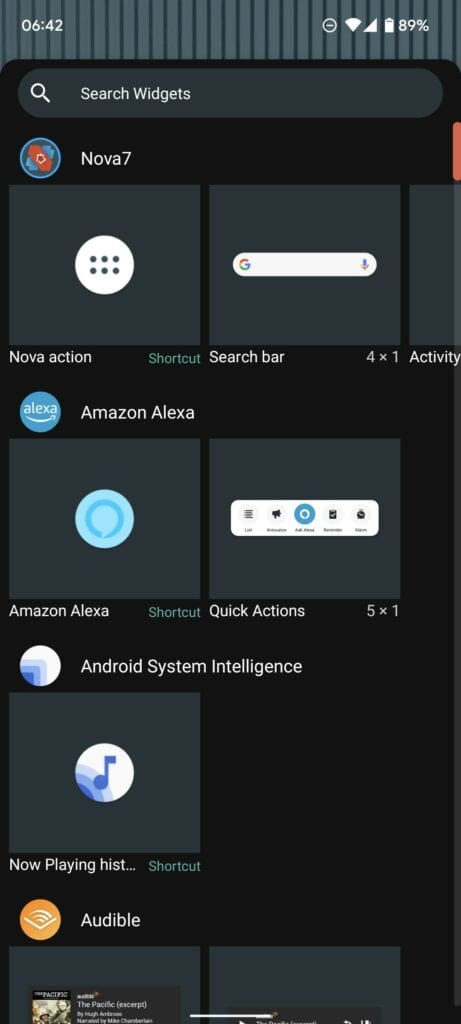The image depicts an Android widget selection screen. At the top, the status bar shows the time as 6:42, a Wi-Fi symbol, a 'Do Not Disturb' icon, full mobile data strength, and an 89% battery level. Below the status bar is a search box labeled "Search widgets." 

The main section displays a list of available widgets. The screen highlights widgets related to the Nova Launcher, a custom launcher for Android, confirming the operating system as Android. The visible widgets under Nova Launcher include "Nova Action," a search bar, and a partially visible one labeled "Activity."

Following the Nova widgets, there are options for Amazon Alexa, including a button to invoke Alexa and a 5x1 widget for quick actions. The "Android System Intelligence" category offers a widget for "Now Playing History," which identifies songs playing in the background. The image also partially shows widgets for Audible, clipped at the bottom edge of the frame.